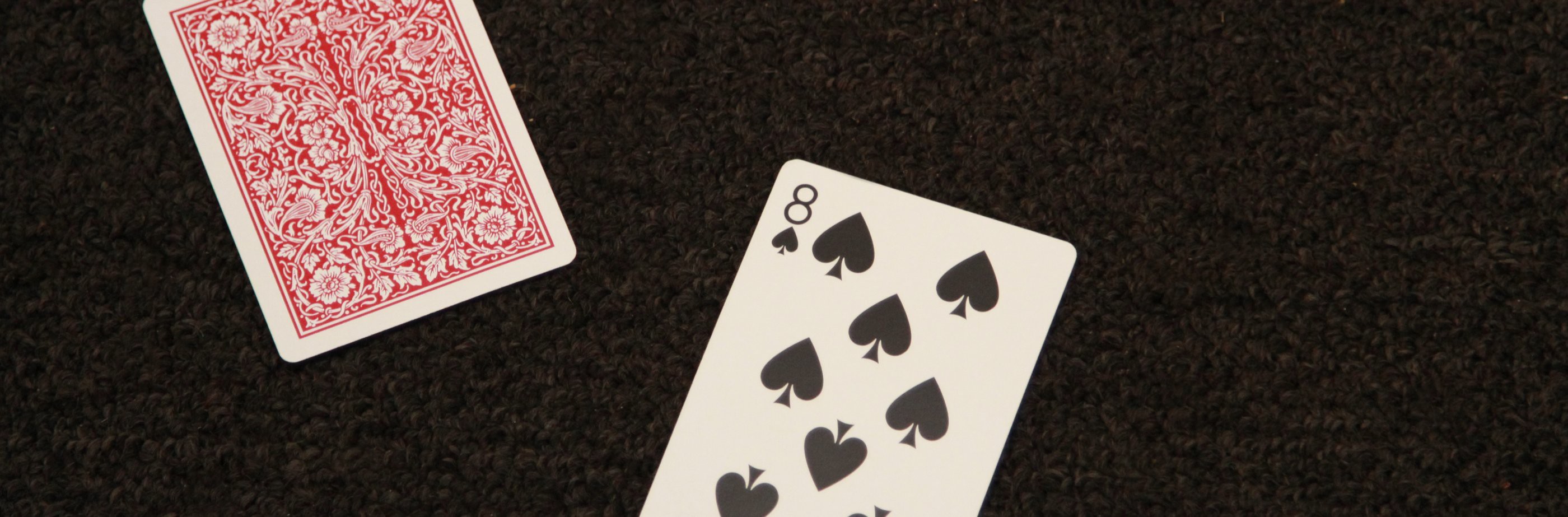This photograph features a sleek, narrow, black rectangular background. Elegantly arranged on this backdrop are two playing cards. Positioned diagonally from the top left to the bottom right, one card displays its intricate back design. The card's edge is white, framing a richly decorative red and white pattern at its center. The design is a harmonious blend of scrollwork, vines, leaves, and flowers, with the crimson hue serving as the background, while the ornate details are rendered in white. 

On the right side of the image, extending from the center towards the top right, is the face of a playing card. This card is easily recognizable as the eight of spades, set against a crisp white background. While seven black spades are clearly visible, the eighth spade is slightly cropped at the bottom right corner of the image. The card's top left corner features a black numeral eight paired with a smaller spade symbol, confirming its identity as the eight of spades without the need to count the individual spades. The overall composition is both striking and meticulously detailed, capturing the viewer's attention with its artistic interplay of design and form.